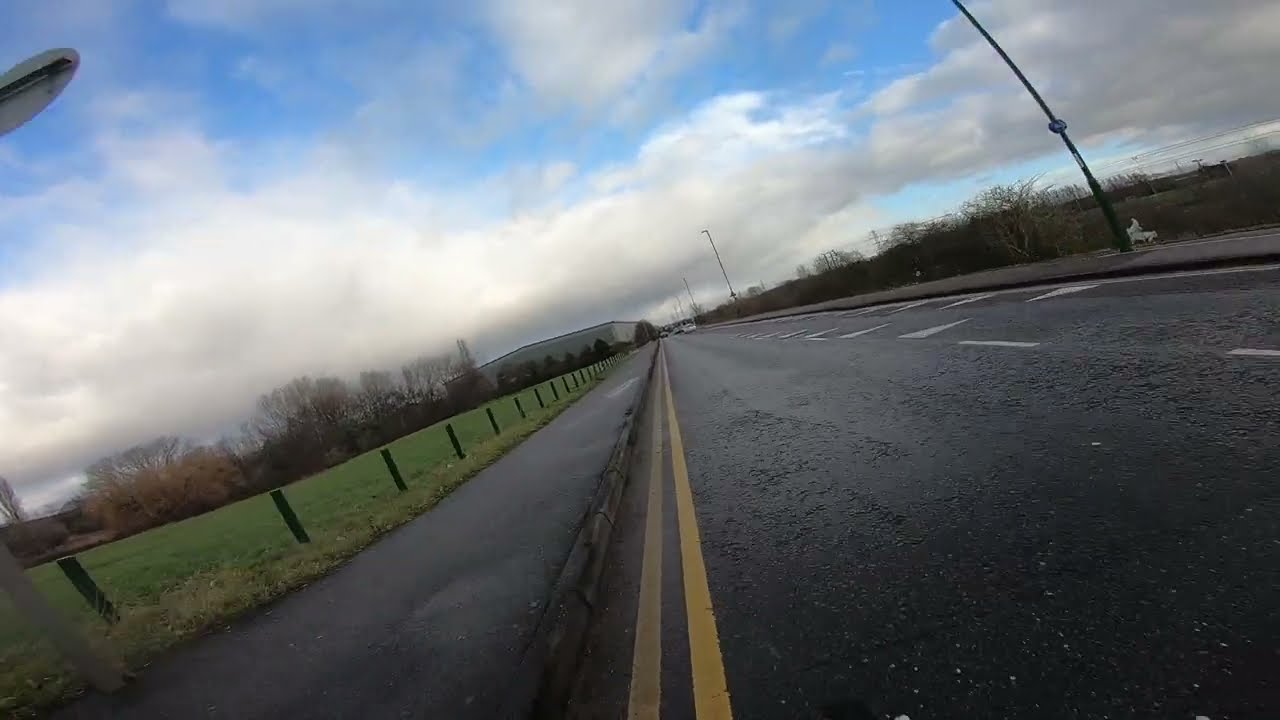This image captures a diagonally slanted view of a major paved road, gently moist from recent rain, evident from its darkened black-gray surface. The scene is set during the daytime under a predominantly cloudy sky with patches of blue. Dominating the center of the image is a double yellow line marking the road. To the left of these lines, there is a sidewalk of the same asphalt material, abutting a grassy area fenced by regular posts. This grassy field extends into the distance with leafless trees and telephone poles, some of which possess sparse yellow foliage. Further beyond, cars can be seen faintly atop the road. On the right side of the road, white street markings stand out against the black asphalt, with light poles sporadically placed along another field. The far background reveals more trees, along with hints of a large white building on the left, culminating this detailed snapshot of a quiet, expansive roadway framed by an overcast sky.